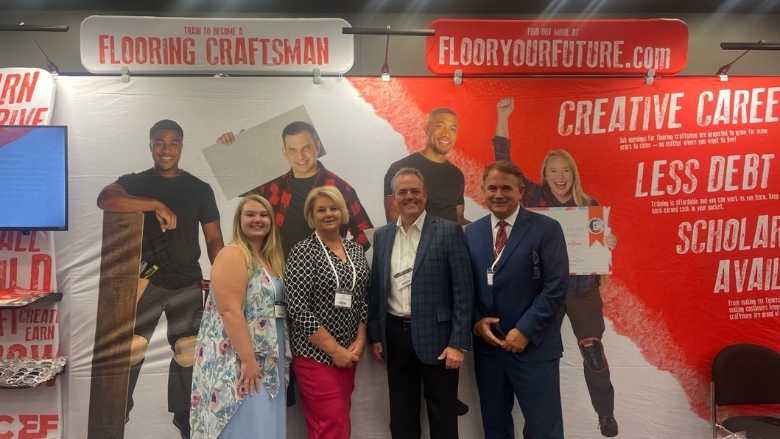The image depicts a group of four Caucasian individuals—two women and two men—posing at a booth in a convention or trade show setting. They all wear name tags on lanyards. The young woman on the far left, possibly in her twenties, is dressed in a long-sleeved dress or coat. Next to her is a slightly older woman with a bob haircut, wearing a black long-sleeve top and red pants. The two men on the right are dressed in business suits; one in a navy suit with a white shirt. They stand in front of a large, red-and-white banner displaying the text "Flooring Craftsman, FloorYourFuture.com" along with a promotional slogan "Creative career, less debt, scholarships available." The banner features images of four enthusiastic young adults holding various materials. All four individuals in the foreground are smiling at the camera.